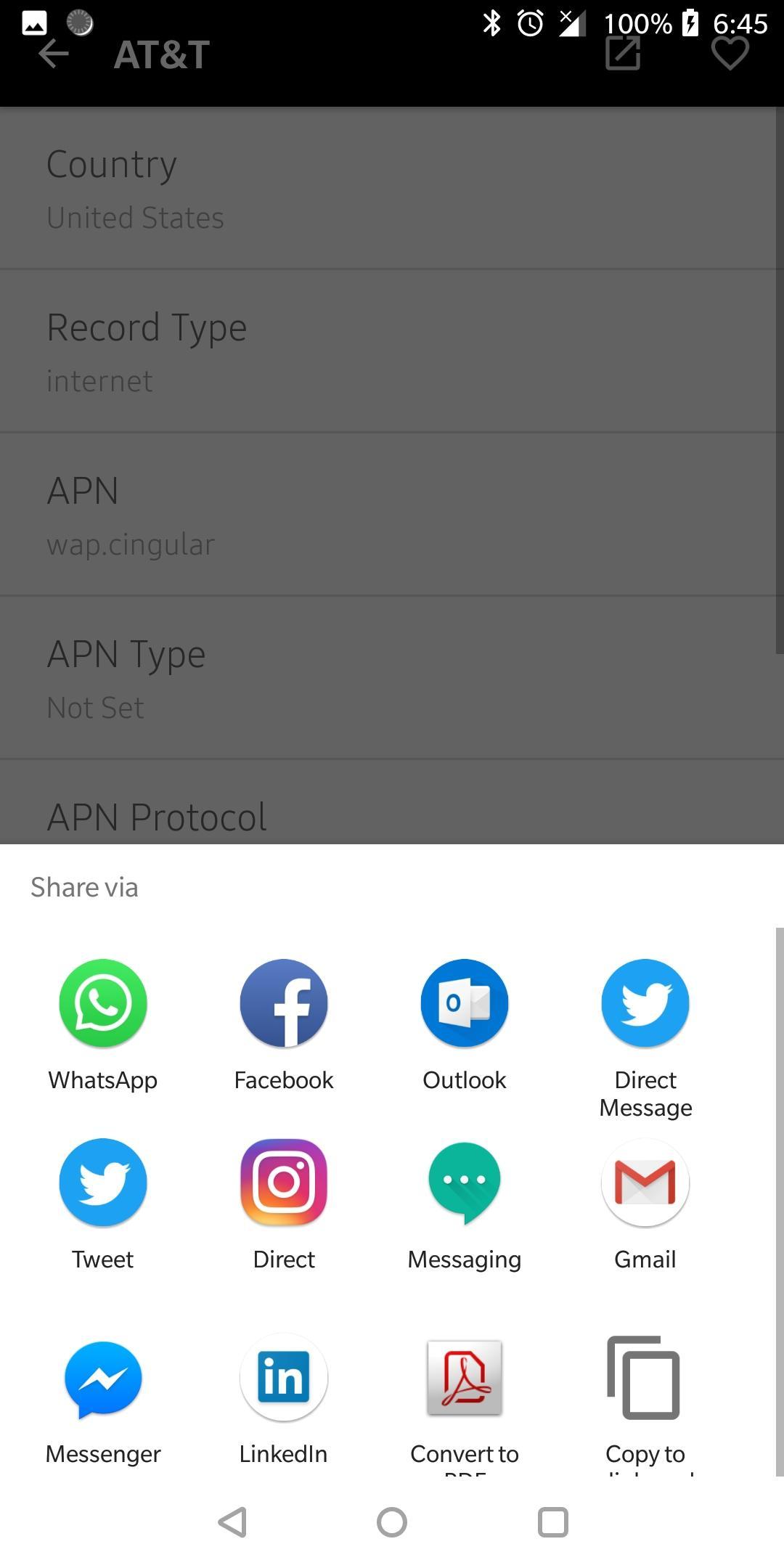The image predominantly features a cell phone screen. The upper portion of the screen is overlaid with a semi-transparent dark gray layer, making it slightly challenging to discern the display. In the top left corner, there's a square icon with a white background depicting two mountains. Moving to the top right corner, several icons can be seen, including the Bluetooth symbol, an alarm clock, and a fully charged battery indicator accompanied by "100%" and "6:45."

Below this, text reads: "Country: United States", "Record Type: Internet", "APN: WAP", "Singular", "APN Type: Not Set", and "APN Protocol." 

The bottom part of the screen, which is not covered by the dark layer, has a white background and contains a section labelled "Share via", followed by a selection of app icons. The apps listed in the first row are WhatsApp, Facebook, Outlook, and Direct Message. The second row includes icons for Tweet, Direct, Messaging, and Gmail. The final row shows icons labelled Messenger, LinkedIn, and two partially visible icons where the text reads "Convert to..." and "Copy to..." but gets cut off.

At the very bottom of the screen, navigation icons are visible: a left-pointing arrow, a circle, and a square.